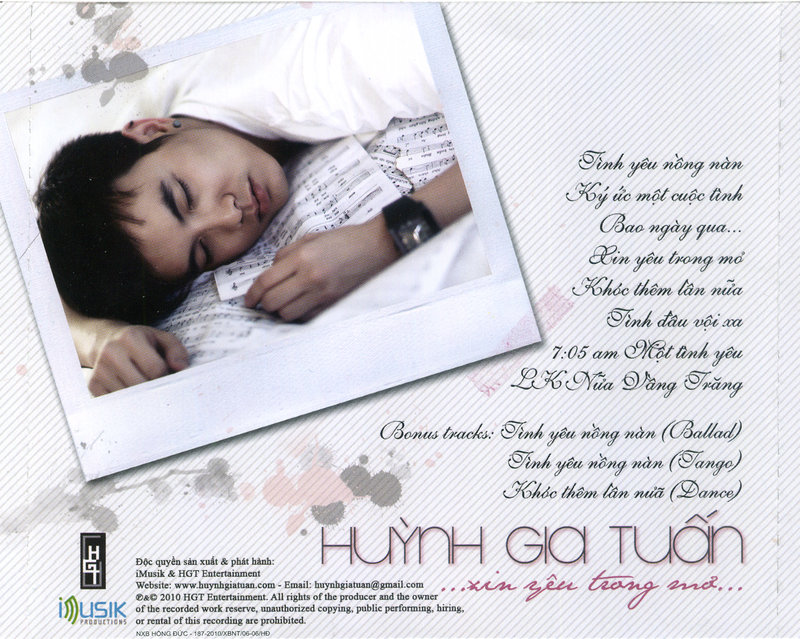The image is an advertisement featuring a light grey striped background with a prominent Polaroid photograph of an Asian man asleep on a pile of sheet music, wearing a white shirt and a black watch, with dark hair. He has an earring in his left ear. This Polaroid appears to be casually pasted onto the background. Adjacent to the photograph are several words in Vietnamese, including "Bonus tracks," "ballad," "tango," and "dance," along with a large title "HUYNH GIA TUAN." Additional text includes "7.05am," implying a possible time of day relevant to the context. At the bottom right, there's a black rectangle box logo with "HG iMusik" and "HGT Entertainment," followed by the website address (www.huynhgiatuan.com) and the contact email (huynhgiatuan@gmail.com). The advertisement also mentions, "2010 HGT Entertainment. All rights of the producer and the owner of the recorded work reserved; unauthorized copying, public performance, hiring, or resale of this recording are prohibited." The official look and details suggest it might be promoting a music album.